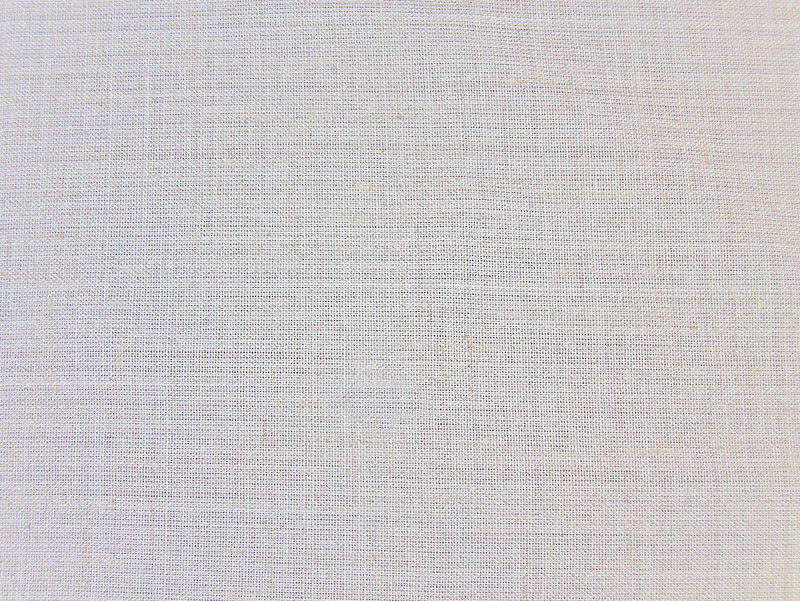This photograph captures an extreme close-up of a fabric, filling the entire frame with a detailed view of its texture. The fabric exhibits a grid-like pattern created by numerous intertwined threads, which appear to vary in color. Predominantly, the threads look off-white or cream, giving an overall light gray hue from a distance. Upon closer inspection, however, subtle variations emerge: some threads display hints of gray, brown, orange, or possibly yellow. The fabric appears somewhat unevenly discolored, particularly towards the right edge of the image, where it may seem slightly darker or even a tad dirty. The threads are not tightly woven, giving the fabric a somewhat loose structural appearance. The image is mostly in focus, though the upper and lower right edges are slightly blurred, adding a sense of depth. As there are no other visible elements, the photograph provides a detailed and concentrated study of the fabric’s texture and color variations.